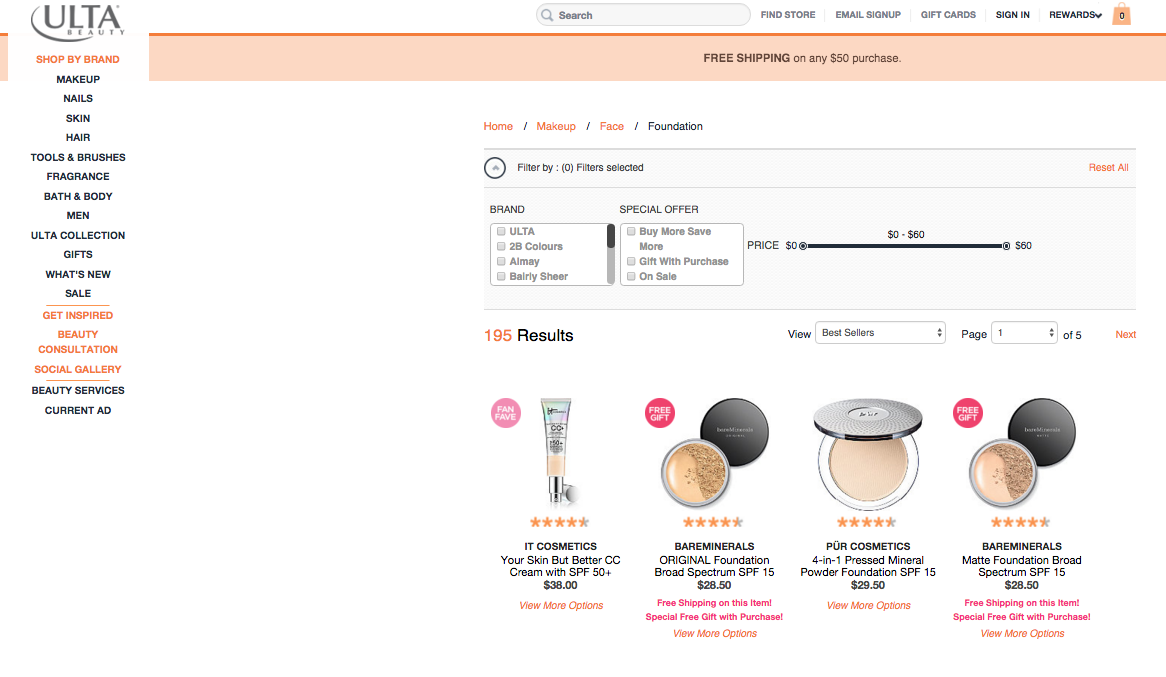Top left of the image features the Ulta logo. Above the displayed items, there's a search bar followed by options for 'Find Store', 'Email Sign Up', 'Gift Cards', 'Sign In', 'Rewards', and a shopping bag icon. Below this navigation bar, there's a prominent red banner advertising "Free Shipping on any $50 purchase."

The main navigation menu below the banner lists categories including: 'Shop by Brand', 'Makeup', 'Nails', 'Skin', 'Hair', 'Tools and Brushes', 'Fragrance', 'Bath and Body', 'Men', 'Ulta Collection', 'Gifts', 'What's New', 'Sell', 'Get Inspired', 'Reality', 'Consultation', 'Social Related', 'Beauty Services', and 'Current Home Makeup Base Foundation'.

Highlighted within the product listings is a special offer promoting 'Buy More, Save More'. The results show 195 items, including 'IT Cosmetics', featuring products like 'Your Skin But Better CC+ Cream with SPF 50+' and the 'Original Foundation by Spectrum'.